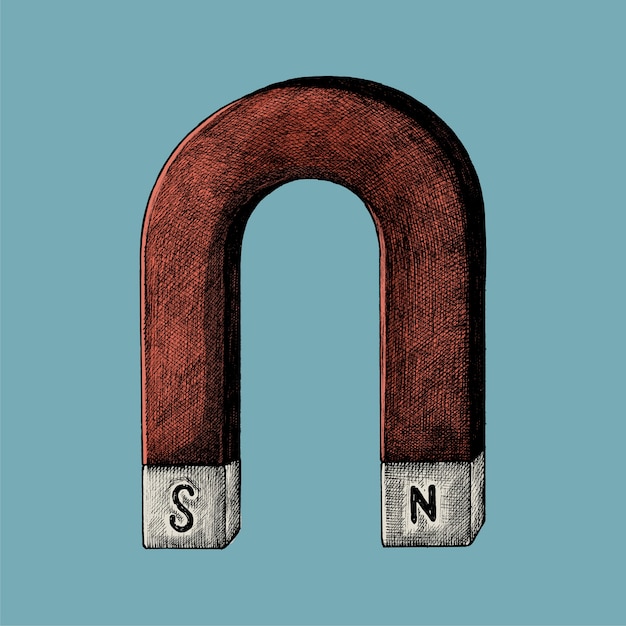This is a detailed illustration of a U-shaped magnet depicted in an upside-down 'U' position. The magnet features a rusty-red hue with meticulously drawn black cross-hatching and pen-stroke shading, which gives it a textured, hand-drawn appearance. The base of the 'U' showcases white tips with cube-shaped ends marked 'S' for South on the left and 'N' for North on the right, each letter appearing engraved into the surface. The background is a teal-blue color, adding contrast and emphasizing the 3D dimensionality of the magnet. The illustration has shadows along both the inner and outer edges of the magnet, further enhancing its depth and realism, though there is no shadow cast beneath it.